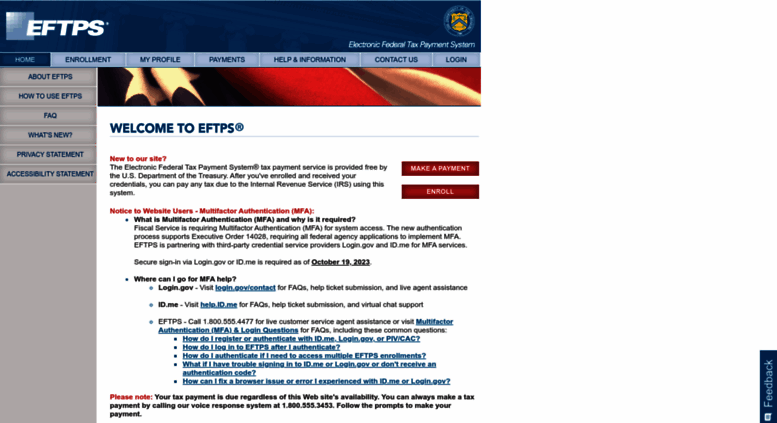The web page features a translucent blue banner at the top, which reveals the upper sections of a classical building adorned with columns. On the left side of the banner, "EFTPS" is prominently displayed in white text, signifying the Electronic Federal Tax Payment System. Adjacent to this, on the right side, is an official badge further reiterating the system's full name.

Beneath the banner sits a lighter blue navigation menu, which turns to the darker shade of the banner when hovered over, revealing a dropdown menu with selectable options. The navigation categories include Home, Enrollment, My Profile, Payments, Self-Information, Contact Us, and Login. Currently, the Home menu is selected, expanding to show six submenu options highlighted in a gray background with blue text.

The main content area begins just below the navigation menu, featuring a truncated image of the American flag at the top. Below this, a warm welcome message, "Welcome to EFTPS," is written in black text against a white background. The page includes various informational sections and is framed on the right by two prominent buttons labeled "Make a Payment" and "Enroll."